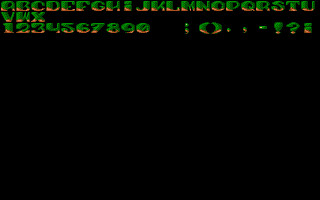Image Description: The image features a black background with green text and symbols. Across the top of the screen, the characters "A, B, C, D, E, F, G, H, I, J, K, L, M, NOP, Q, R, S, T, U, V, W, X, 1, 2, 3, 4, 5, 6, 78, 90" are displayed in an orderly fashion. Beneath this sequence, there is punctuation including a semicolon, a period, a comma, a dash, an exclamation mark, and a question mark. The terms "banana" and "mirrored banana" are also present in the text. Additionally, there is an icon resembling a pill bottle with a brown dash across the bottom. All the mentioned characters and icons are rendered in green, maintaining a consistent color scheme. The brown dash at the bottom adds a contrasting element to the predominantly green and black composition.